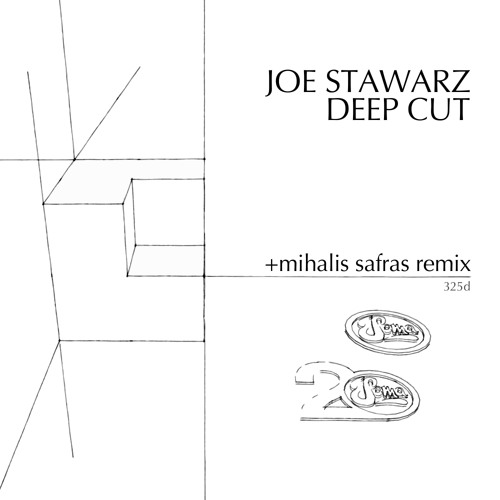The image is a minimalist black and white album cover, featuring thin, angular geometric line patterns predominantly on the left side. In the upper right-hand corner, the text reads "Joe Stawars" followed by "Deep Cut," and just below it, "Plus Mihalis Sofras Remix, 325D" is inscribed horizontally. The lower right-hand quadrant of the cover includes two hand-drawn emblems; the first one is a rounded circle with the word "SUM," and directly below it, a similar emblem with the phrase "2 in SUM." The overall design is very simple and sparse, emphasizing clean, intersecting, and parallel lines which create a structured, cubist style. The entire cover is rendered in stark black and white, with the background in white and the lines and text in black.